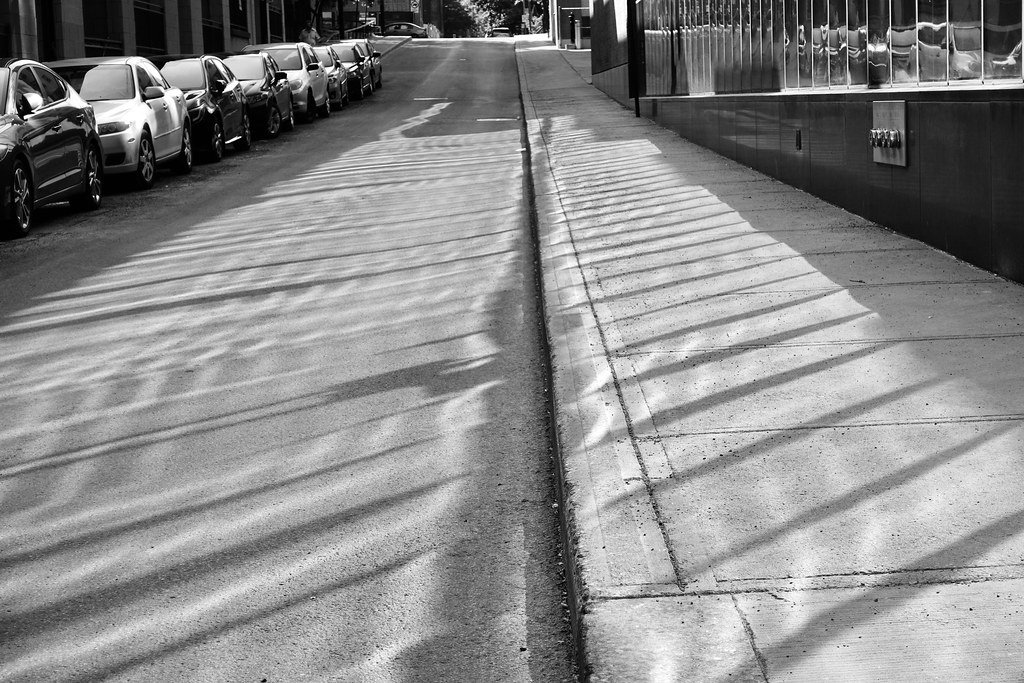This black-and-white photograph captures a detailed urban scene from a city neighborhood. The image is taken from a close-up vantage point on a sidewalk, which runs alongside a two-lane street. On the left, eight cars are neatly parked along the curb, their forms clearly visible against the stark monochrome backdrop. The road itself is devoid of any moving vehicles, emphasizing the stillness of the moment. Shadows cast by the sunlight create a play of light across the scene, with the light reflecting sharply off the building windows on the right. This building, adjacent to the sidewalk, features multiple windows with mirrored surfaces that catch and reflect the sunlight. Beyond the immediate foreground, the street and sidewalk gradually narrow and rise over a small hill before dipping downwards, leading the eye towards a distant background dotted with a few trees. The overall impression is one of quiet urban elegance, marked by the careful composition of architectural elements and natural light.